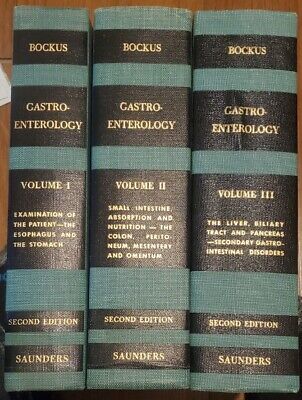This photograph showcases the spines of three upright, hardcopy medical books against a beige-brown background. The image, presented as a vertical rectangle, focuses entirely on the book bindings, which are predominantly teal and black with gold lettering. Each book spine is designed with alternating black and teal horizontal stripes, featuring five black sections separated by teal lines. The text on the black sections is gold.

The first book on the left reads "Bacchus Gastroenterology Volume 1: Examination of the Patient, The Esophagus and the Stomach, 2nd Edition, Saunders." The middle book states "Bacchus Gastroenterology Volume 2: Small Intestine, Absorption and Nutrition, The Colon, Peritoneum, Mesenteries, and Omentum, 2nd Edition, Saunders." The book on the right says "Bacchus Gastroenterology Volume 3: The Liver, Biliary Tract and Pancreas, Secondary Gastrointestinal Disorders, 2nd Edition, Saunders." All three books are part of the same series with consistent styling, emphasizing the meticulous categorization of gastroenterology topics.